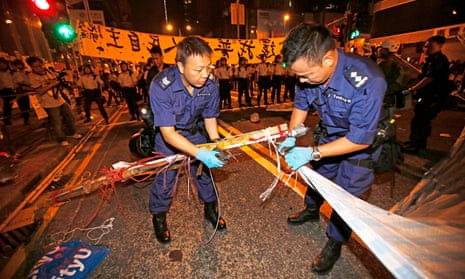The nighttime photograph depicts a street scene, presumably in an Asian country such as China, with two men in the foreground and a large crowd in the background. The two men, who appear to be wearing blue uniforms—possibly police or armed forces uniforms—are engaged in assembling or modifying a long bamboo stick. One of the men is tying ropes to the bamboo stick while the other is attaching a white piece of cloth to it. Both men are wearing blue latex gloves, short blue pants, black shoes or boots, and have short dark hair. Behind them is a large, illuminated banner with Chinese characters. The area is filled with individuals dressed in white shirts and black pants, possibly uniformed, some wearing helmets. The street is notably devoid of vehicles, further suggesting it has been closed off, and the scene is washed in the orange glow of street lights and traffic signals, enhancing the night-time atmosphere. Cameramen are visible amidst the crowd, capturing the event.